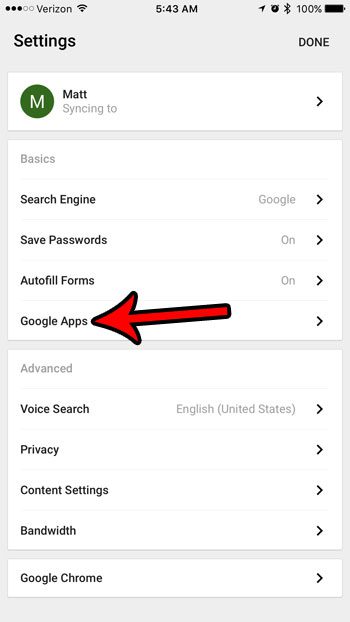The screenshot showcases the settings page of a mobile device with a white background. At the upper left corner, the word "Settings" is prominently displayed. Below this, a green circle with a white "M" is visible, next to the name "Matt." Beneath Matt's name, the text "Sinkin2" appears in gray. Further down, options listed in gray include "Basics," "Search Engine," "Save Passwords," "Autofill Forms," and "Google Apps." A red arrow specifically points towards "Google Apps." Toward the lower part of the screen, additional settings are shown, with "Advanced" written in gray. The options listed in black under "Advanced" are "Voice Search," "Privacy," "Content Settings," "Bandwidth," and "Google Chrome."